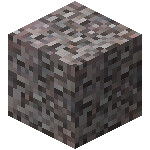The image depicts a highly pixelated digital block from the popular video game Minecraft, characterized by its distinct cubical shape and intricate pattern of small, square pixels. These pixels create a textured surface composed mainly of varying shades of gray, black, and brown, giving it a rocky, cobblestone-like appearance. The block is oriented with one corner facing the viewer, allowing for a clear view of three of its sides – the front, the left, and the top. This detailed visualization showcases the uniformity across its faces, maintaining the same pixelated pattern throughout. Easily recognizable to those familiar with Minecraft, this block typifies the game's signature building materials and embodies the game's iconic, digitized aesthetic.